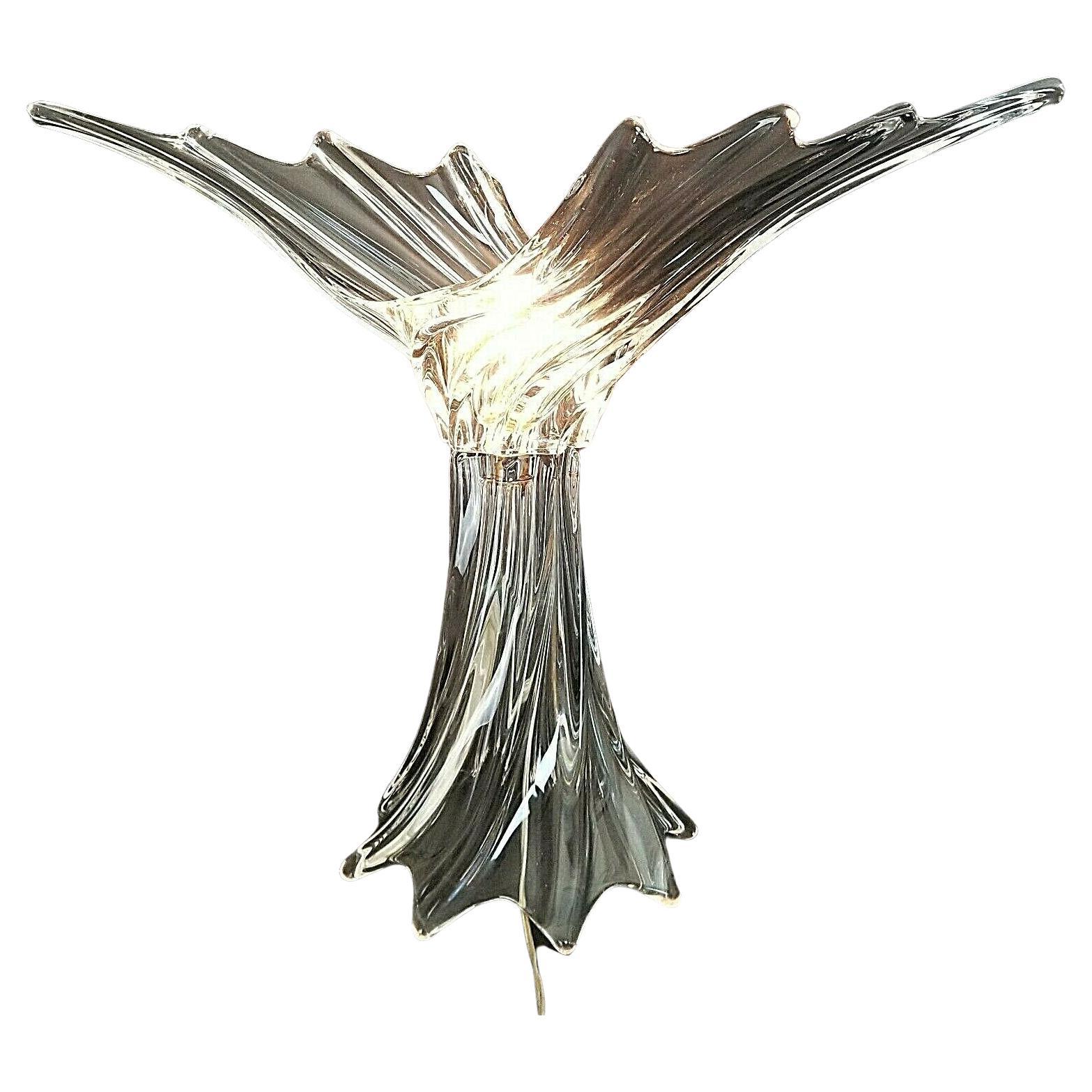The image features a sophisticated and unique piece of home decor, possibly a stand-up lamp designed for display or sale. The background of the image is completely white, highlighting the intricate object in the center. The lamp, resembling a vase, stands prominently adorned with colored glass. At its base, the lamp showcases a dark gray hue, while towards the top right, it transitions into a brownish color. 

A visible power cord runs from the middle of the lamp down to the bottom, suggesting its functionality as a lamp. The material appears to mimic stainless steel, with a polished, metallic finish, although it might actually be high-quality plastic painted to give a stainless steel look. The base of the lamp resembles a tree trunk, which branches out in an organic and flowing manner, reminiscent of waves in water. The light source seems to be located in the middle, indicated by a bright yellow glow that gradually transitions into a brownish color as it moves outward from the center. 

The lamp's structure includes three distinct sections: upper left, upper right, and a central downward section. Each section is designed to reflect or emit light, creating an elegant and polished aesthetic. This lamp is not only a functional lighting piece but also a piece of art, with its shiny, clean, and expensive appearance making it a standout piece in any setting.